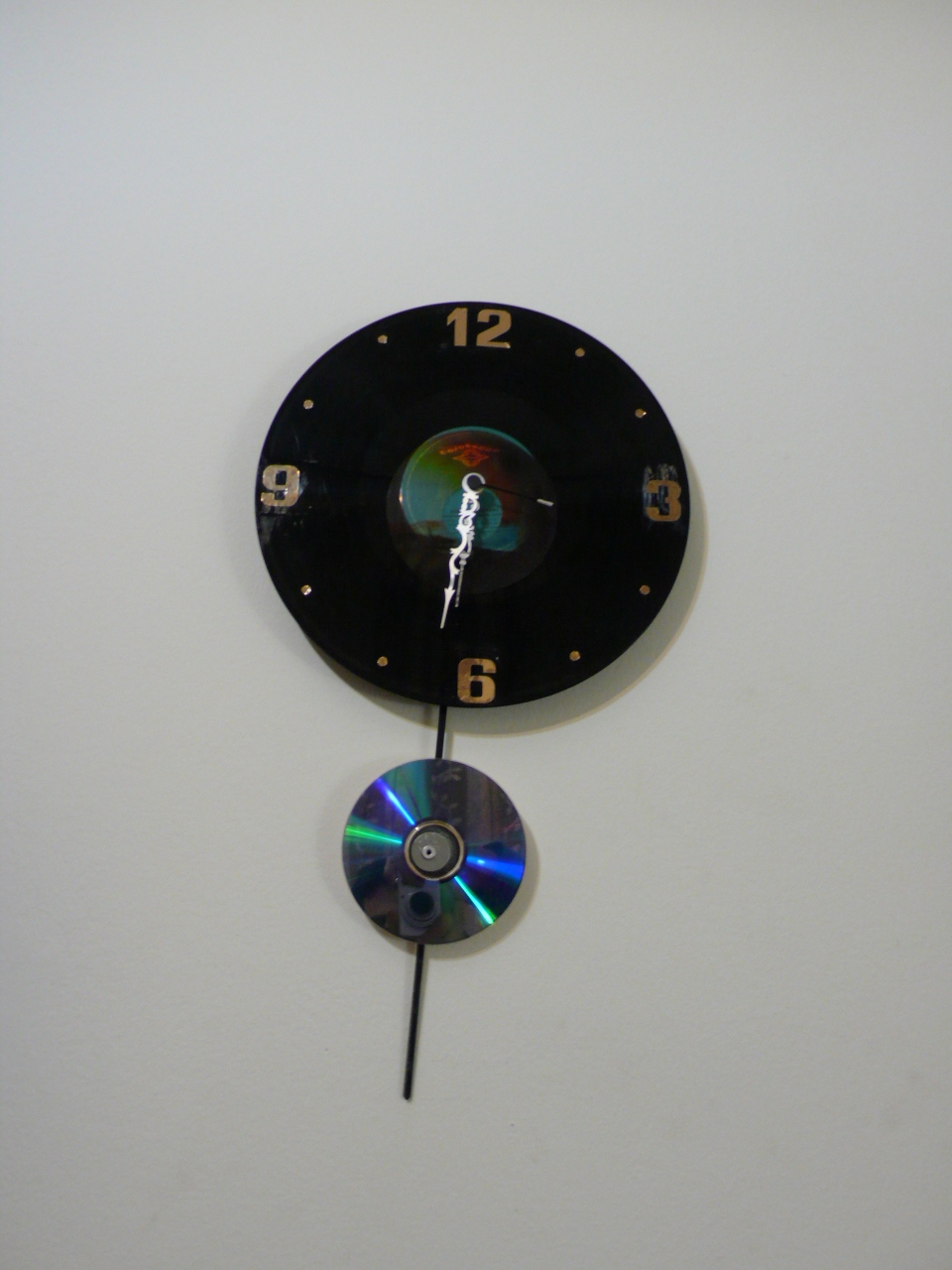The image depicts a photograph of an analog clock mounted centrally on a plain, off-white, perhaps slightly gray wall due to the lighting. The clock itself resembles a black vinyl record, circular in shape. Its face includes the gold numbers 12, 3, 6, and 9 at the corresponding points, with small gold dots marking the remaining hours. The clock has white hands, indicating a time of approximately 6:30. The label at the center of the clock is mostly obscured but appears to have a teal background with a gradient of blue, orange, and red mixed with some light green and brown. A distinctive feature of the clock is a pendulum-like element beneath it, described as the underside of a burnable CD with a shiny, reflective surface displaying light reflections in hues of blue and green. This reflective surface also captures part of the photographer's hand and their small digital camera.